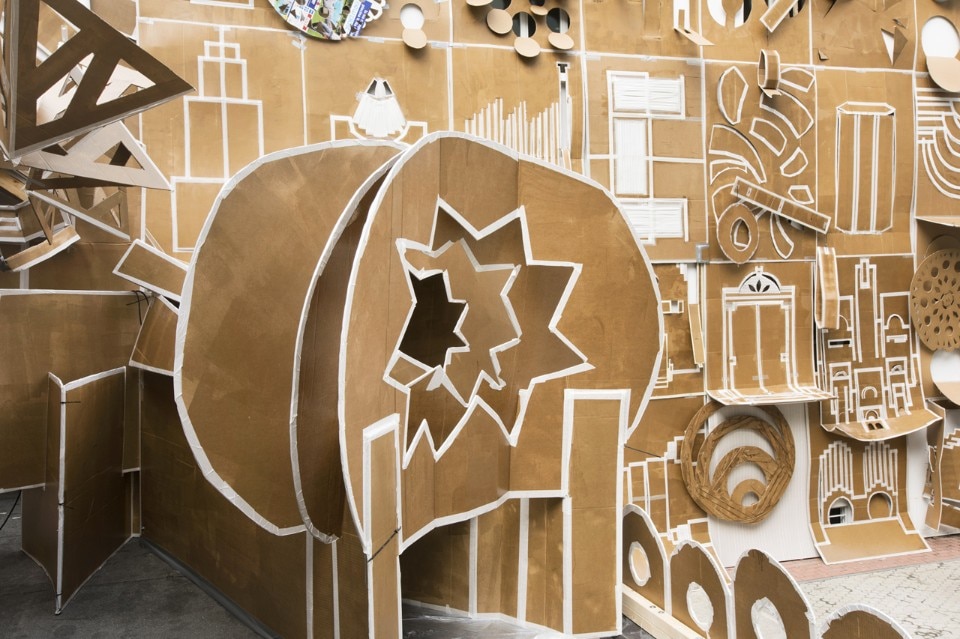The photograph captures an art exhibit showcasing a monochrome display dominated by shades of brown and white. The walls of the room are adorned with large rectangular sections of thick, brown, cardboard-like paper, each bordered in white and featuring intricate geometrical designs. Among the shapes, there are diamonds, circles, and spheres, mixed with representations of buildings and hands. Each design appears to be meticulously cut out of heavy-duty black and white paper. The exhibit also features a central three-dimensional structure that resembles a small tunnel or passageway, creating a sense of depth and movement. This striking and detailed composition, reminiscent of recycled grocery bags, juxtaposes simple and complex forms, inviting viewers to explore its wild, wacky, and imaginative spatial elements.